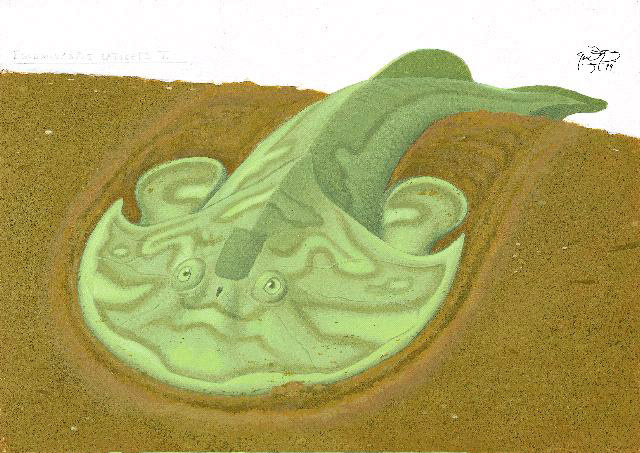The illustration depicts a fantasy sea creature emerging from the water onto dark, sandy terrain. The creature, painted in varying shades of green from pea soup to mint, features a body reminiscent of a trilobite or horseshoe crab with a human-like, gargoyle face. Its eyes protrude like a flounder's, set above a small, nose-like hole and a lined smile. The creature's tail is pointed, with a small upright fin on its back and additional fins behind its head, which resembles ears. The sandy foreground is a blend of brown and gold hues, while the background is stark white. Brown lines and intricate patterns add detail to the creature's form. In the upper right corner, an artist's signature with initials and date is visible, although partially obscured. On the upper left, there is faint, unreadable text suggesting a title.